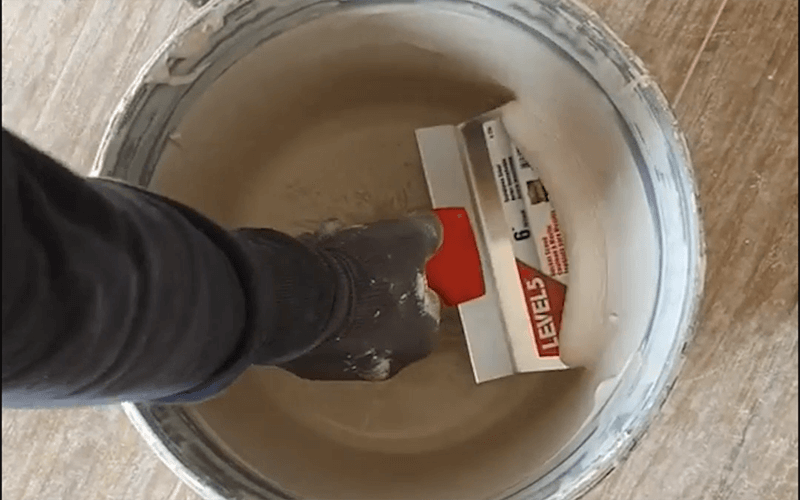In the image, there is a close-up of a workman scraping the remaining white, creamy putty from a heavily used paint can. The person is wearing a long, dark grey sweatshirt and thick, charcoal black gloves speckled with white paint. The tool they are using appears to be a spatula or a similar device, featuring a red handle and a stainless steel scraping end, with a partially visible label reading "Level 5." The paint can itself is grey with dried paint around its rim, indicating extensive prior use. The scene is set on a distressed, greyish oak wood floor, which surprisingly lacks any protective covering, even though the work involves potentially messy materials. The workman is meticulously trying to scoop out and reuse the last of the thick, white putty, which is likely intended for smoothing drywall seams. The detailed setup and the condition of the tools suggest that the task is essential and the materials are being conserved carefully.